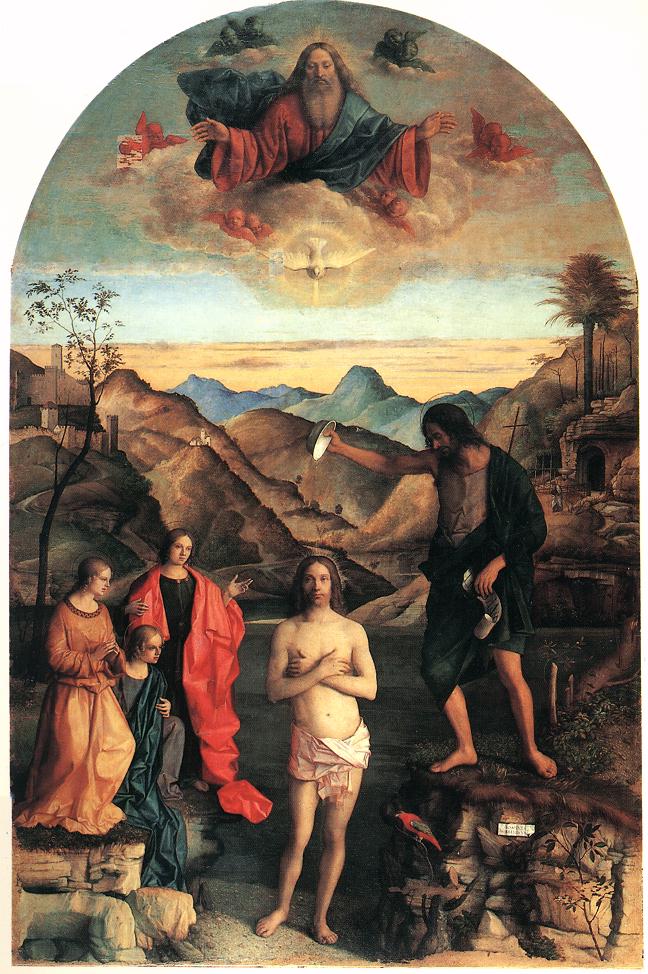The painting depicts a biblical scene rendered in a cylindrical pattern with rich, dark colors. At the top of the image, a divine figure resembling God, distinguishable by his long flowy brown hair, white beard, and red robe with a blue or green shawl, gazes down from the heavens. He is surrounded by angels in hues of red, black, and green, and enveloped in clouds, with a white dove subtly positioned beneath him, signifying the Holy Spirit.

Below the celestial scene, the ground transitions into a field and then rolling brown mountains adorned with small huts and trees. In the foreground, five central figures are set against this rugged landscape. Three women stand on the left, each distinct in their attire: one wears a coffee brown robe, another a teal gown, and the third a black dress accented with a red shawl. 

Central to the scene is a half-naked man, modestly covered with a cloth around his lower body, his arms crossed over his chest. He exudes an aura suggestive of Jesus Christ. To his right, another man stands atop a rocky platform, barefoot, clad in a partial green garment. This person appears to be pouring liquid from a bowl over the half-naked man, possibly signifying a baptismal act. The overall composition and detailed elements strongly suggest a religious narrative, possibly an allegory or depiction of a sacred ritual.